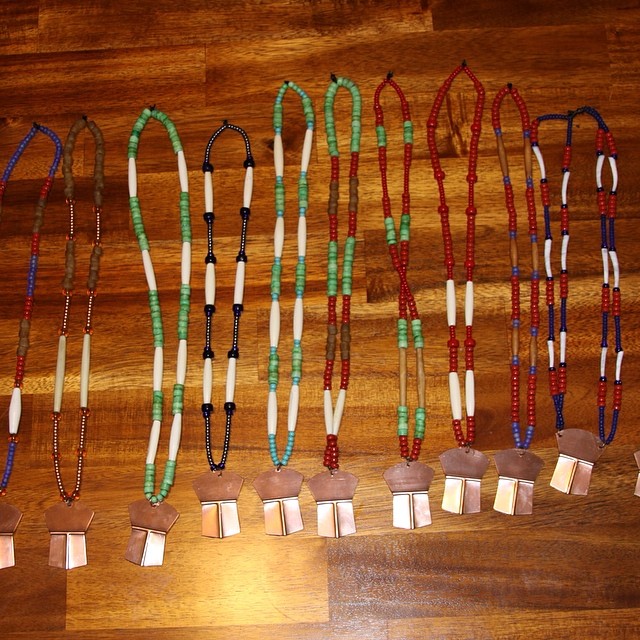In this detailed image of ceremonial beaded necklaces, the scene is set against a rich, wooden background that varies from golden brown to dark brown hues. The photograph, taken directly from above, captures about 10 to 12 necklaces hanging from small black hooks. These necklaces, tribal in nature, are adorned with vibrant beads in colors such as bright dark red, deep blue, lighter blue, white, green, and black. The beads are strung along the entire length of the necklace, creating a pattern reminiscent of puka shell designs. Each necklace features a distinctive brass-colored pendant at the end, shaped somewhat like a half-moon with an abrupt cut-off, leading to a square-like middle that protrudes slightly. The overall lighting in the image is concentrated towards the bottom, casting a subtle shadow and creating a gradient effect towards the top.